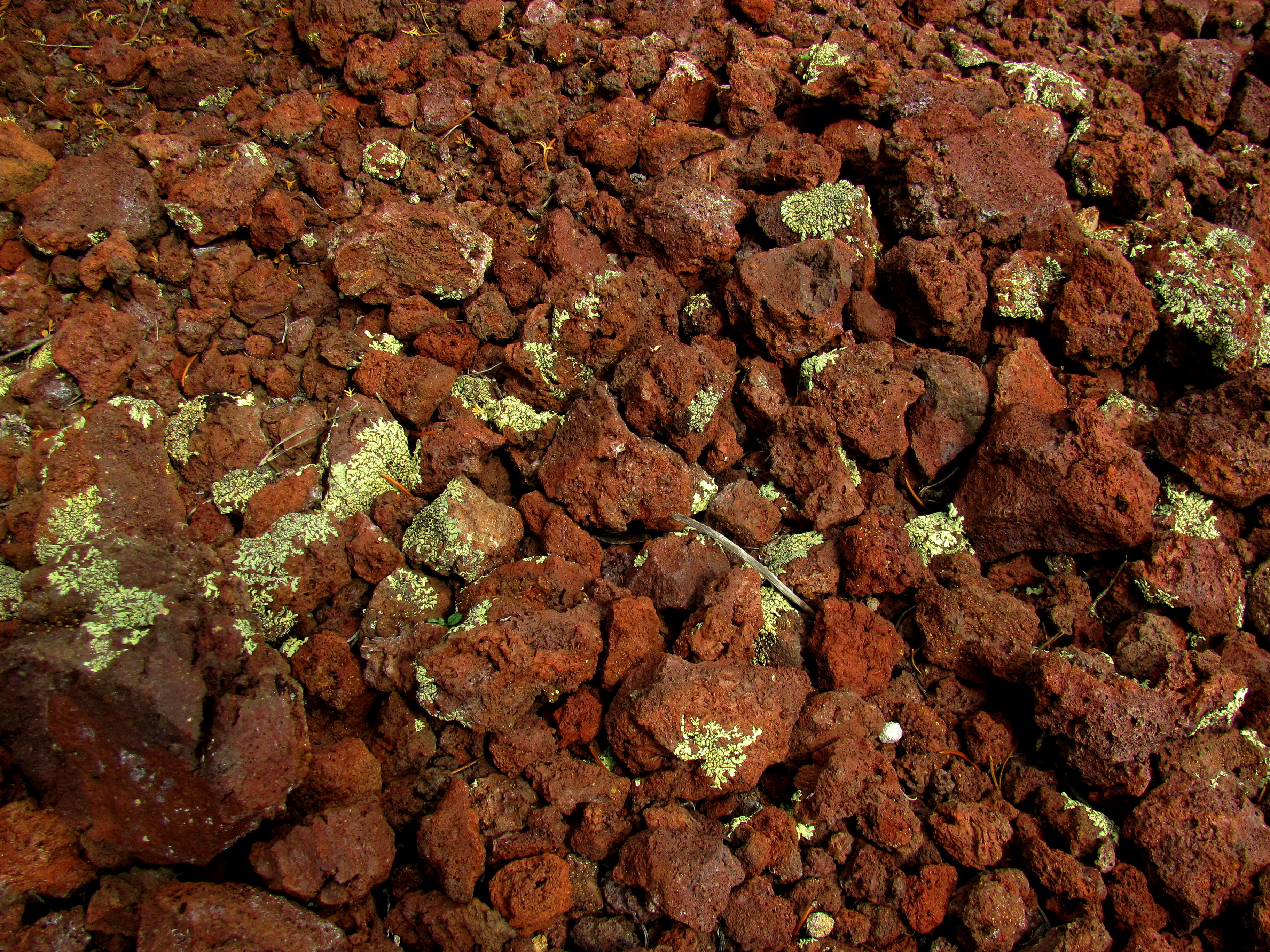This is a detailed close-up photograph showing a sprawling bed of rocks of varying sizes and shapes, viewed from above. The rocks predominantly exhibit a deep, dark reddish color mixed with hues of orange and brown. Speckled across several rocks are light-colored portions ranging from whitish-green to yellowish-tinted moss or fungus growths, highlighting the natural textures. Some rocks appear tiny, reminiscent of pebbles, while others are as large as baseballs, contributing to the diverse array of dimensions within the image. The scene possibly depicts broken clay bricks, given the reddish clay-like appearance of the stones. Despite some ambiguity about the exact cause of their fragmentation, whether due to natural processes or mechanical intervention, the image conveys a rich, earthy tableau bathed in broad daylight, with a slight yellow tint enhancing the overall illumination.